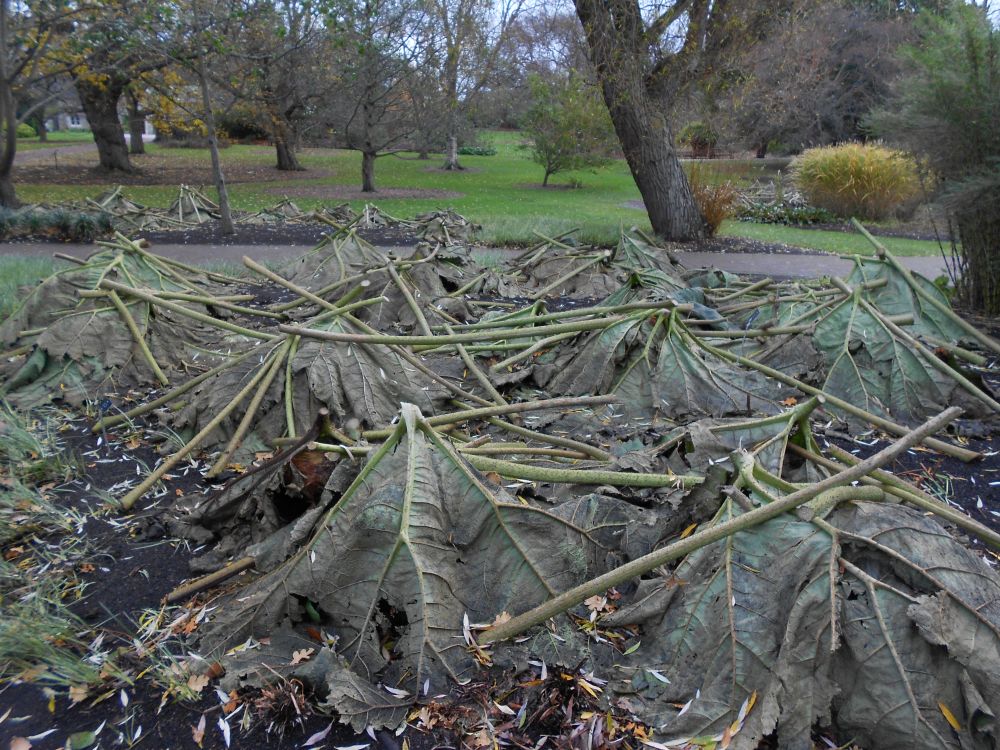A detailed photograph captures an intriguing scene on a bright, potentially cloudy day. The image is dominated by large, tent-shaped leaves on the ground, arranged face down in a pattern reminiscent of shallow teepees. The dull green leaves show triangle-shaped veins and brown, crunchy edges, indicating decay. They appear to be elephant ear leaves, broad and about the size of a hand. These leaves seem to cover piles of smaller leaves and are possibly held in place by cut branches, about an inch or two in diameter.

The bottom half of the image reveals rich, dark soil with small grass blades and finer leaves scattered around. To the left, small tufts of grass cling to life, while to the right, a small green bush adds to the landscape. A sidewalk cuts through the scene beyond the leaves, leading to a large, bright green park or public space. Several trees with thin trunks and green to yellow leaves dot the grassy plane, contributing to the serene environment. Towards the farther right, a fluffy green bush and a large yellow bush punctuate the scene, anchored by a background building. The well-maintained trees and vibrant grass suggest a well-cared-for area, contrasting with the decay and arrangement of the leaves in the foreground.